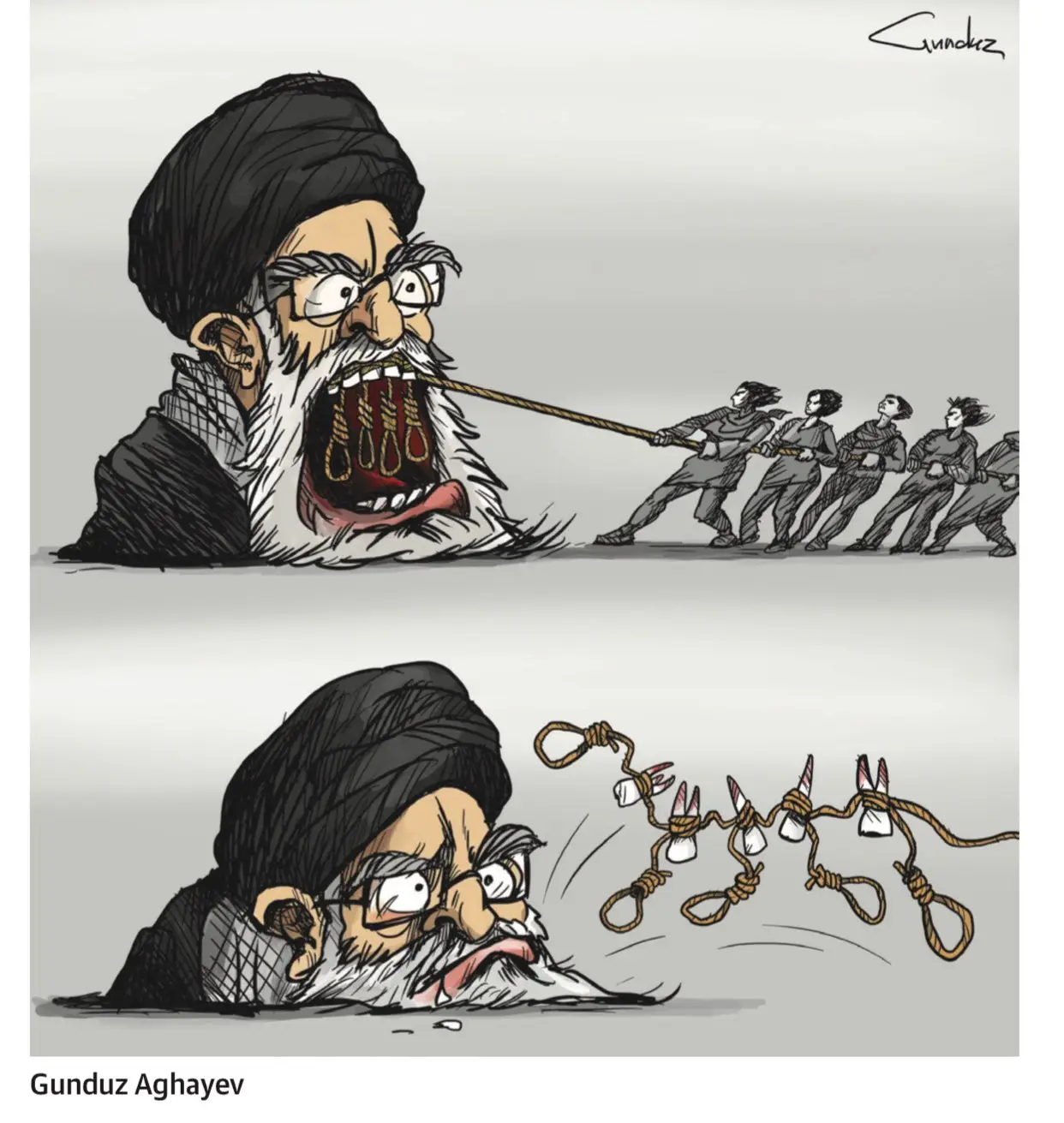The image is a political cartoon by Gunduz Aghayev (G-U-N-D-U-Z A-G-H-A-Y-E-V), as indicated by the signatures placed at the top right and bottom left of the artwork. The cartoon is presented in two panels. The top panel features an elderly, bearded Iranian mullah, characterized by his black head wrap, turban, and glasses. His mouth is wide open, and ropes are wrapped around his teeth, forming nooses. Five individuals are depicted in a tug-of-war stance, pulling these ropes with all their might. In the bottom panel, the mullah's mouth is closed and his chin rests on the ground as if in defeat. His teeth, now dislodged, are visible flying through the air still attached to the ropes. The imagery suggests a dramatic extraction of power or voice, highlighting a significant political message.